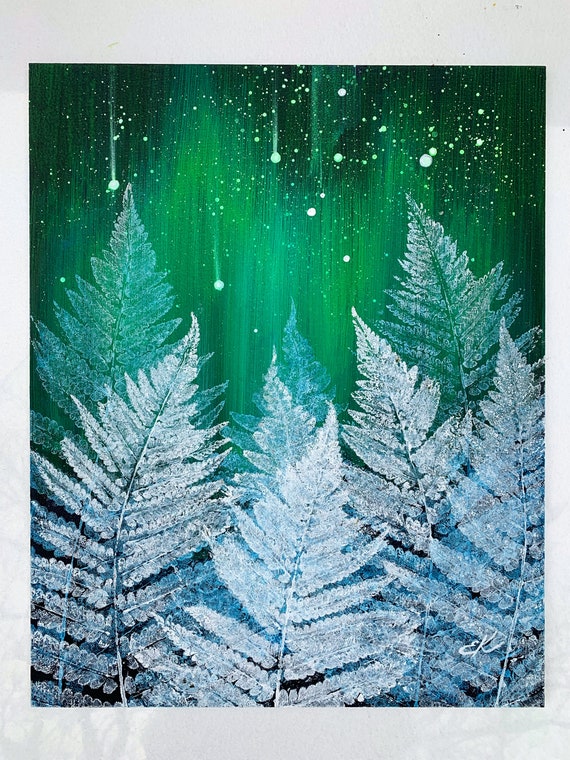The image is a beautifully detailed artistic representation, appearing either printed, stamped, or painted. It portrays a serene Arctic or sub-Arctic scene dominated by fern-like leaves that also resemble snow-covered trees. These leaves, primarily white with shades ranging from snowy white to medium blue and deeper turquoise, are layered and slightly curved at the tips, all pointing vertically upwards. The background, reminiscent of the Northern Lights or aurora borealis, features fluid, zigzagging streaks of green in various shades, creating an ethereal atmosphere. Scattered throughout are white speckles, some resembling falling snow or shooting stars, adding to the wintry feel. A light gray border frames the scene, about an inch thick at the top and half an inch on the sides. The initials "EK" are delicately inscribed on the lower right, indicating the artist. This image captures a peaceful, cold weather landscape with intricate details and a captivating sky.